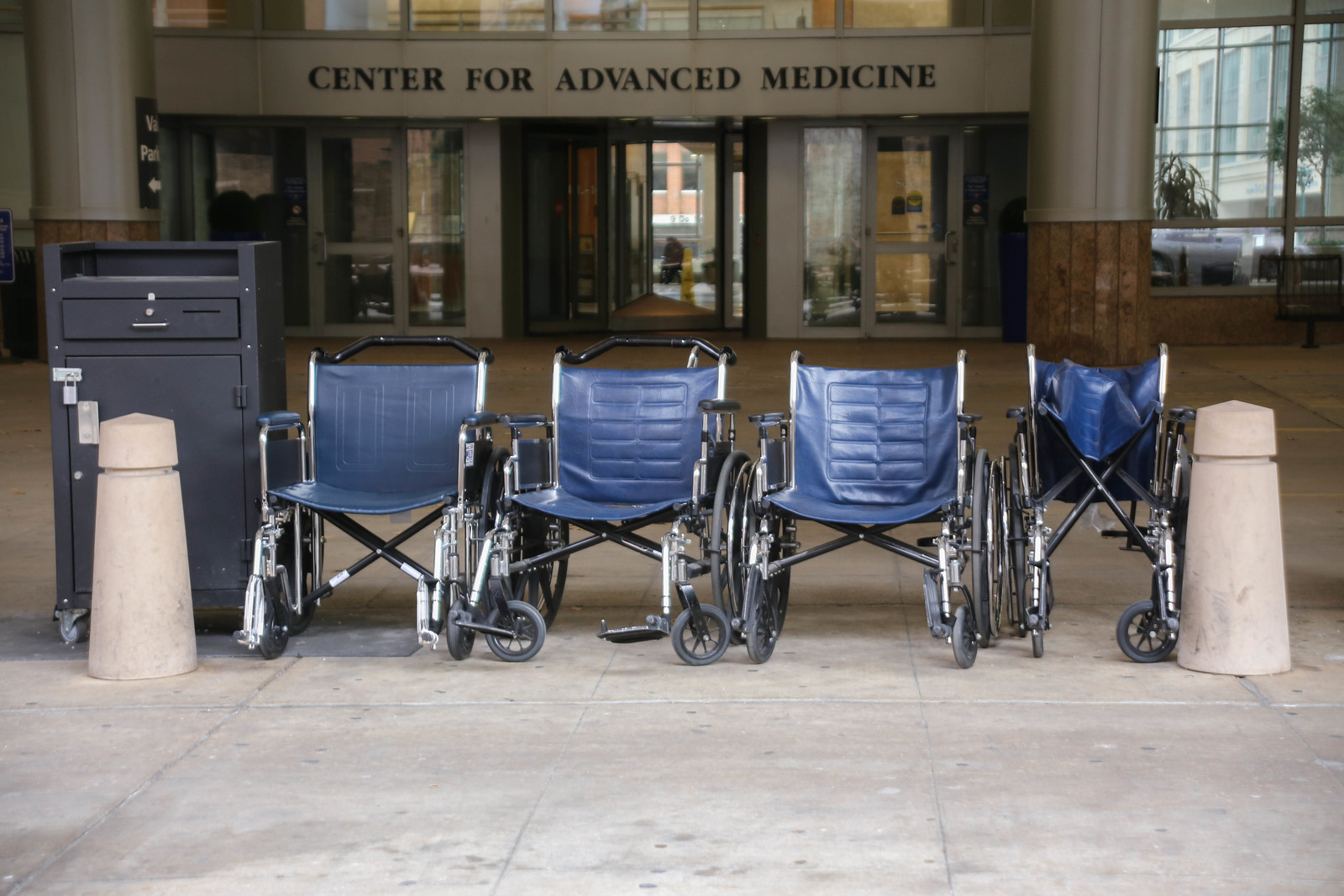In the outdoor daylight photograph, we see an entrance to the "Center for Advanced Medicine," clearly marked in bold black capital letters over the doorway. The building features a central revolving door flanked by two manually openable side doors. In front of this entrance, four unoccupied blue wheelchairs with metal frames are lined up on the concrete sidewalk, facing directly towards the camera. One of these wheelchairs on the far right is partially collapsed. The scene is framed by two stone pillars, one of which has a black valet parking sign attached, and behind one pillar there is a black stand resembling a portable podium or a holder for valet keys. The background, slightly darker than the foreground, includes reflective windows and additional architectural details of the medical facility. There are no people visible in this photograph, contributing to a calm yet somewhat clinical atmosphere.